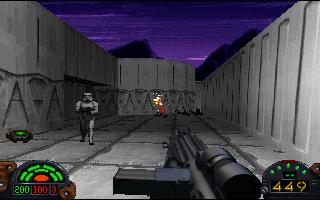In this horizontal, landscape-oriented image from a video game, we find ourselves immersed in a first-person shooter, likely a Star Wars game. The scene unfolds in a narrow, gray-walled alley with a hint of a purple sky and silhouetted mountains in the background. Central to the image is a powerful-looking gun with a large round barrel and a black sight, held by the player in the foreground. The gun appears to be discharging orange sparks or blasts towards a fully armored white stormtrooper further down the alley, who is aiming back at the player. To the right of the gun, a yellow number 449 likely indicates the remaining ammunition. Additionally, there’s a meter on the right side with green and red indicators, showing values of 200 and 100 respectively, accompanied by green lights above it. This image vividly captures the intensity of the moment as the player navigates through a hostile environment.